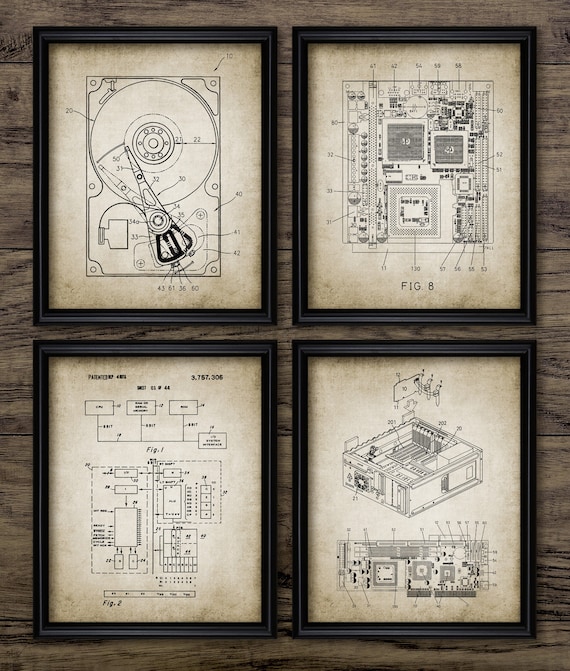The image showcases four identically-sized black rectangular picture frames, each containing what appears to be vintage blueprints of various technological items. These frames are arranged neatly on a black, wooden surface. The top left frame displays a blueprint featuring a large round circle indicative of a machinery part, possibly a CD player, and is annotated with numbers ranging from 10 to 60. In the top right frame, there's a schematic resembling a motherboard, labeled "Figure 8" at the bottom, with numerical annotations throughout. The bottom left frame contains another vintage blueprint, somewhat difficult to decipher, but clearly labeled with numbers including 3, 757, 206, and identified as "Figure 2." Lastly, the bottom right frame presents what seems to be a PC blueprint, illustrating the back of a computer with labeled components and instructions for part placement. Each frame's paper has a distinct aged effect, adding a historical touch to the overall presentation.